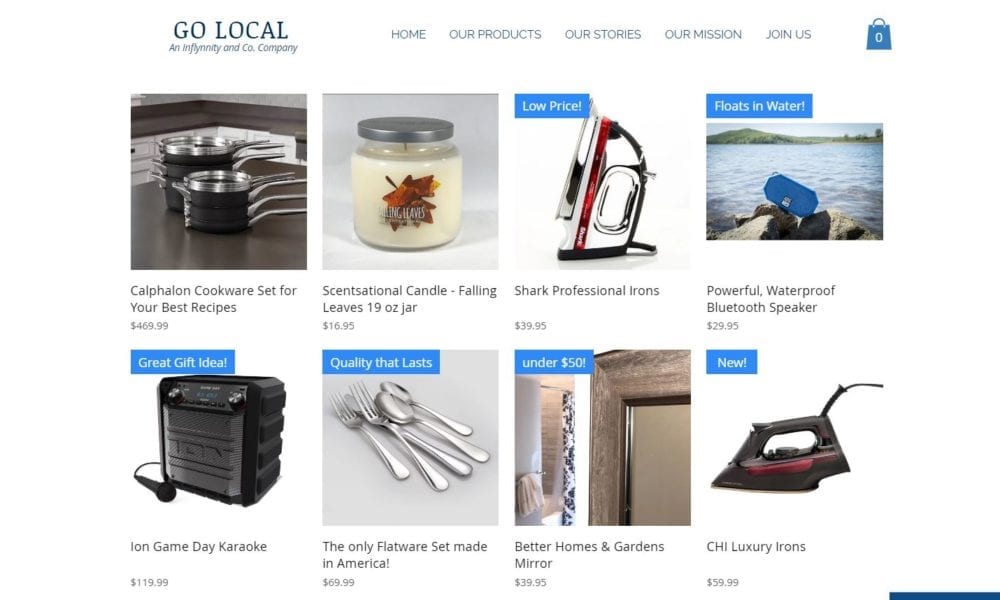Screenshot of a Cropped Web Page

The screenshot captures a cropped web page with a simple, white background. At the top left corner, the page title reads "Go Local" and is branded with "Infinity & Co." On the right side of the header are categories listed in blue font: "Home," "Our Products," "Our Stories," "Our Mission," and "Join Us." Adjacent to these categories is a blue icon of a shopping bag.

Below the header, the main content features a grid of product thumbnails, arranged in two rows with four thumbnails per row. Each thumbnail includes a product image, title, and price, formatted uniformly.

Starting from the top left:

1. A thumbnail displaying a set of pots and pans labeled "Kaplan Cookware Set for Your Best Recipes" priced at $469.99.
2. To the right, a thumbnail of a partially burned candle titled "Sensational Candle Falling Leaves 19 Oz Jar" priced at $16.95.
3. Next, a thumbnail featuring a side view of an iron displays a banner at the top left corner that reads "Low Price" in blue, with the title "Shark Professional Irons" priced at $39.95.
4. The last thumbnail in the first row shows a Bluetooth speaker with a banner that states "Floats in Water."

The second row follows the same format, each featuring a product thumbnail with its respective title and price.